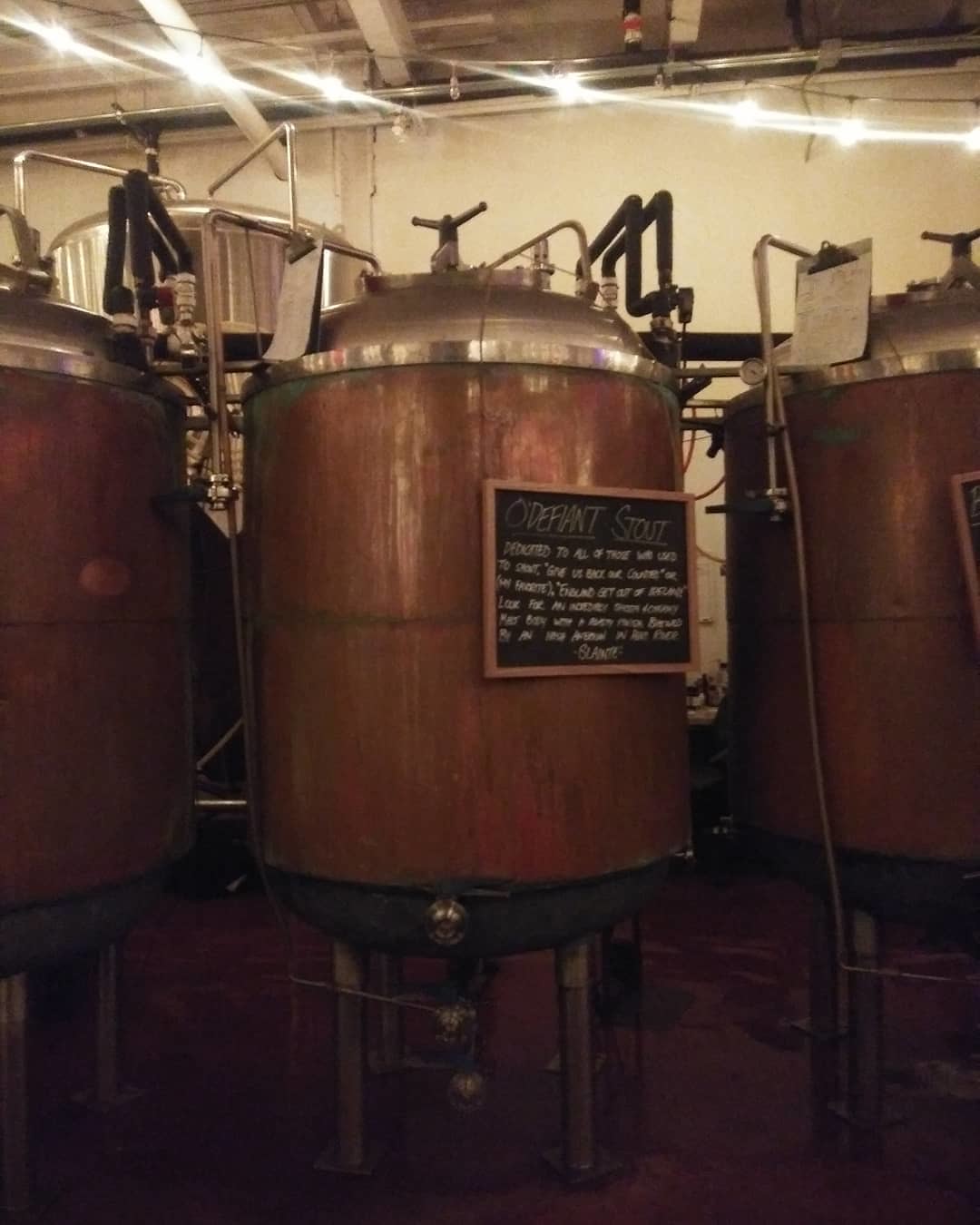Inside a large, industrial brewery, a photo captures an impressive, sizable beer-making operation featuring three prominent copper brewing vats. These large vessels, elevated on sturdy legs, dominate the scene. Each vat is adorned with round, silvery chrome lids equipped with central stopcocks and detailed pipework running in and out, underscoring the complex brewing process. 

The central vat stands out with a blackboard, framed in brown, attached to it. Written in chalk, the readable portion of the sign proclaims "O-Defiant Stout," hinting at the type of beer being crafted, while additional, smaller text remains undecipherable. 

On either side of the central vat, partial views of two similar tanks are visible, contributing to the symmetric layout. The environment exudes an industrial feel, highlighted by the high ceiling with white rafters and hanging, bright ceiling lights. The background also reveals numerous pipes interwoven along the ceiling, enhancing the space's functional aesthetic.

Completing the scene, the brewery's walls are painted off-white, and the floor appears to be a dark red, reinforcing the industrial yet artisanal atmosphere of this vibrant craft brewery.